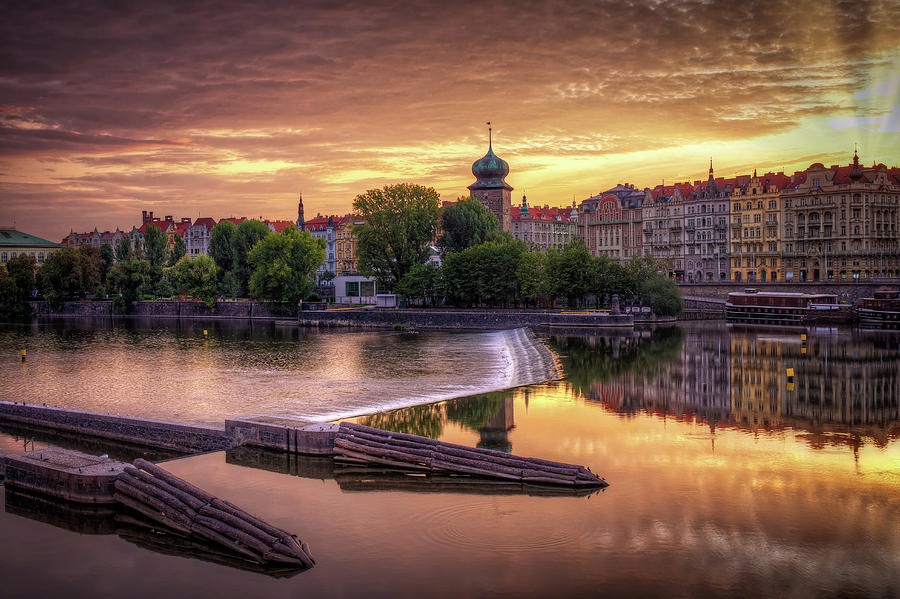The photograph captures a serene European cityscape with a calm, glass-like waterway and a man-made dam featuring a small, three-step waterfall in the foreground. The water perfectly mirrors the sky, which is painted with hues of pink, red, orange, and gray as the sun sets, casting a warm glow across the scene. On the right side of the river, small boats can be seen, adding a touch of activity to the tranquil setting. The banks of the river are lined with green and yellow trees, juxtaposing the urban elements with a hint of nature. Propped against a concrete barrier near the dam are bundles of logs or sticks, adding rustic charm to the otherwise urban landscape. In the background, the cityscape features tall, multi-leveled buildings with classic European architecture in shades of red, yellow, and off-white, topped with distinct red roofs. The old-fashioned buildings stretch across the horizon, providing a picturesque skyline that reflects the rich cultural tapestry of the city. The overall composition is enhanced by the sunset’s light, which creates a harmonious color scheme and a compelling reflection in the water.